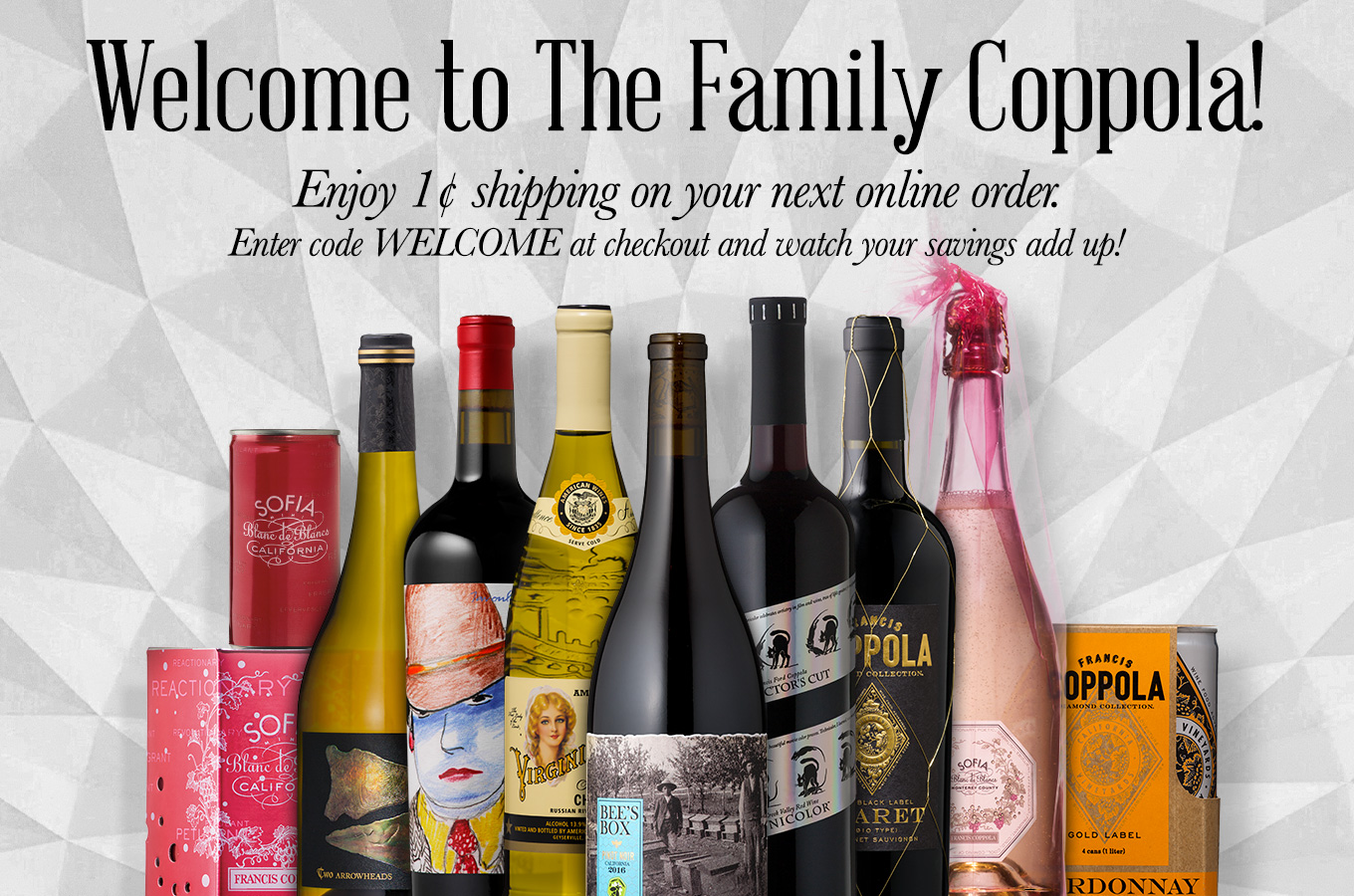The color photograph serves as an advertisement for Coppola beverages, featuring a prominent display of various canned and bottled drinks positioned at the front. The background is adorned with a gray and white fan-shaped triangle pattern. Bold black text at the top welcomes viewers with "Welcome to the Family Coppola!" followed by a promotional message, "Enjoy one cent shipping on your next online order. Enter code WELCOME at checkout and watch your savings add up."

On the left side of the image, several red cans with white text bear the name "Sophia." In the center, a variety of wine bottles are showcased, each adorned with distinctive graphic labels. One notable label "Bee's Box" features a black-and-white photograph of a standing man. To the right of these bottles, more beverages are displayed, including an orange can with black text that reads "Coppola."

This advertisement effectively highlights the diverse range of products offered by the Coppola brand, artistically arranged and detailed to entice potential customers.